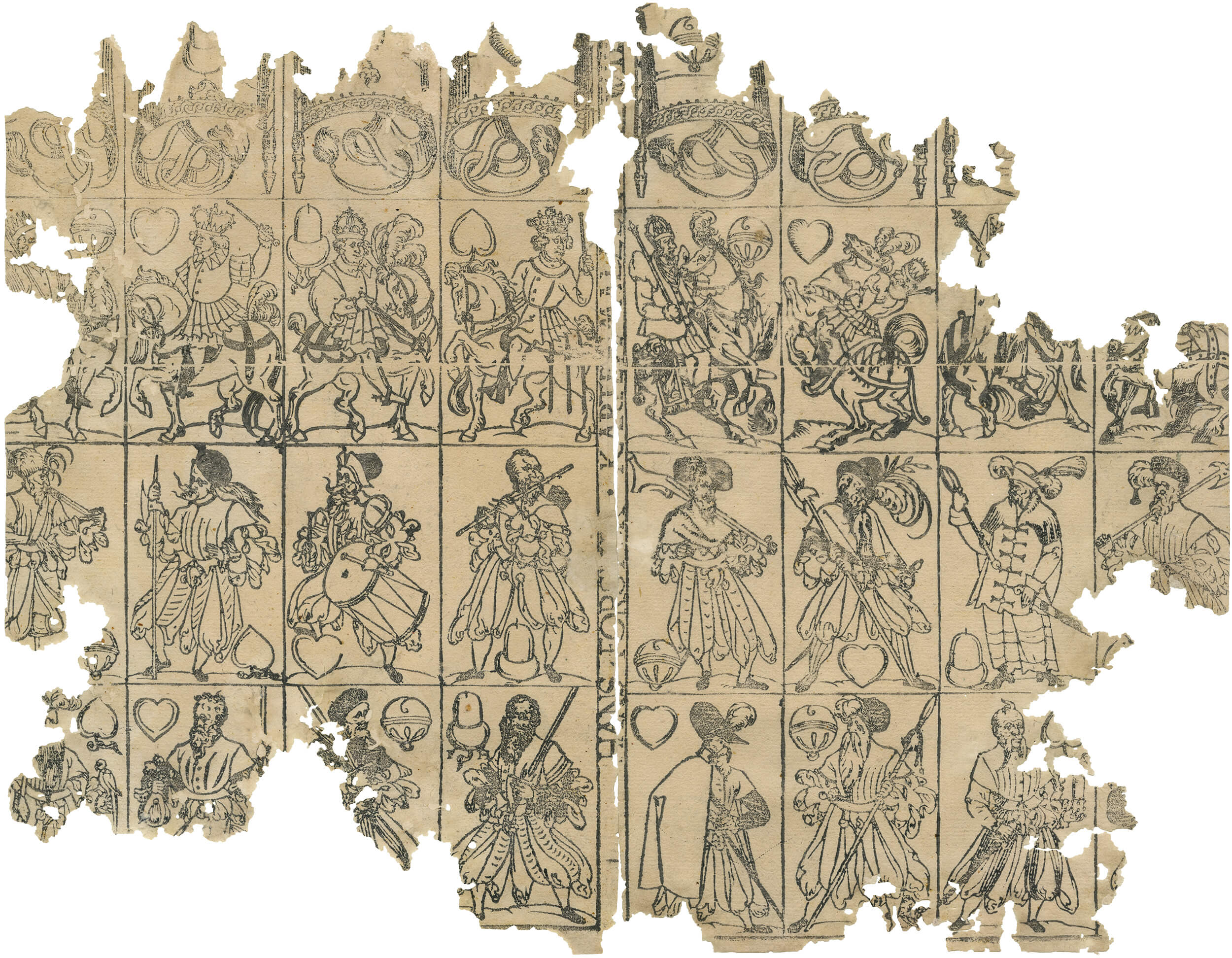The image features two highly tattered pieces of ancient parchment against a pure white background. Each paper, resembling brown, weathered material perhaps once used as wallpaper or part of a medieval text, is laid out flat and divided into rectangles defined by black ink lines. These rectangles contain intricate black ink illustrations of medieval characters and scenes, resembling an uncut deck of cards. The overall condition of both pieces is extremely poor; the edges are irregular and fragmented, giving an impression of a worn-out map. The left chunk is nearly intact, showing pictures of soldiers, riders, musicians, and robed figures possibly resembling kings in sequential rows. The right chunk is more torn, with much of the contents faded or missing, yet still hints at grand medieval imagery. The detailed illustrations and their arrangement into rows evoke the look of an ancient comic strip or storyboard.